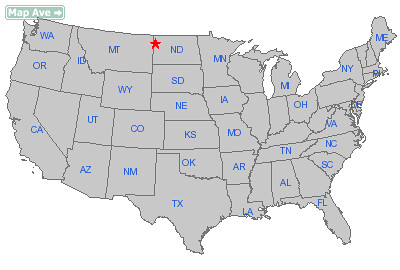The image is a digitally generated clip art-style map of the continental United States. The entire map is in gray, with each state labeled by its two-letter abbreviation rendered in blue. The state borders are depicted with pixelated red lines. Notably, a red star is marked on North Dakota, between Montana and Minnesota. In the upper left corner of the image is a green traffic sign featuring a white right-pointing arrow and the text "MAPAV" in white letters.